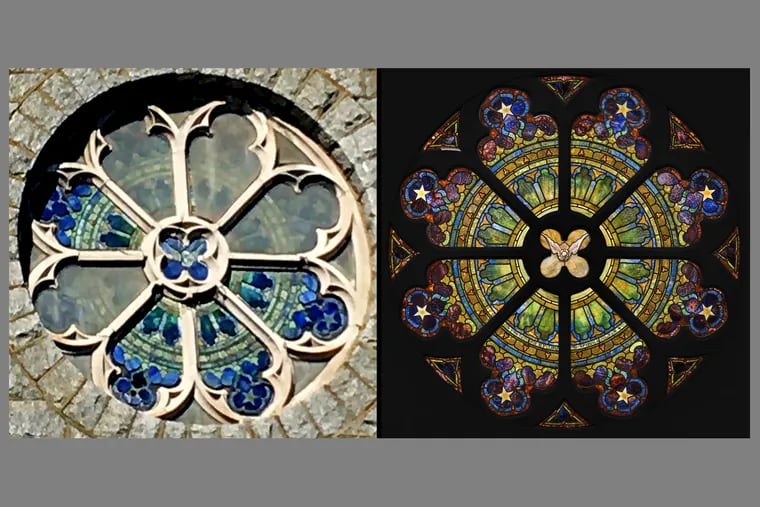The image depicts a side-by-side comparison of a stained glass window during daytime and nighttime. It is framed within a horizontal rectangle with gray borders along the top, bottom, and sides. The window, set in a stone building, features an elaborate circular design reminiscent of a flower with an array of petals. The left image, taken during daylight, reveals a mostly white, metal flower shape with seven or eight petals, some of which contain patches of blue stained glass, while others remain clear. The centerpiece is a smaller circle with four petals, also holding some blue glass. The right image, captured at night, dramatically enhances the stained glass's vibrancy. The same flower pattern now bursts with colors including greens, browns, blues, purples, and reds, accentuated by intricate yellow stars on the tips of the petals. The complex arrangement consists of a green center surrounded by concentric rings of yellow, brown, blue, and yellow again, culminating in blue circles with yellow stars at the petal endings. The detailed and remarkable transformation from daytime to nighttime underscores the window's artistic and structural intricacies.